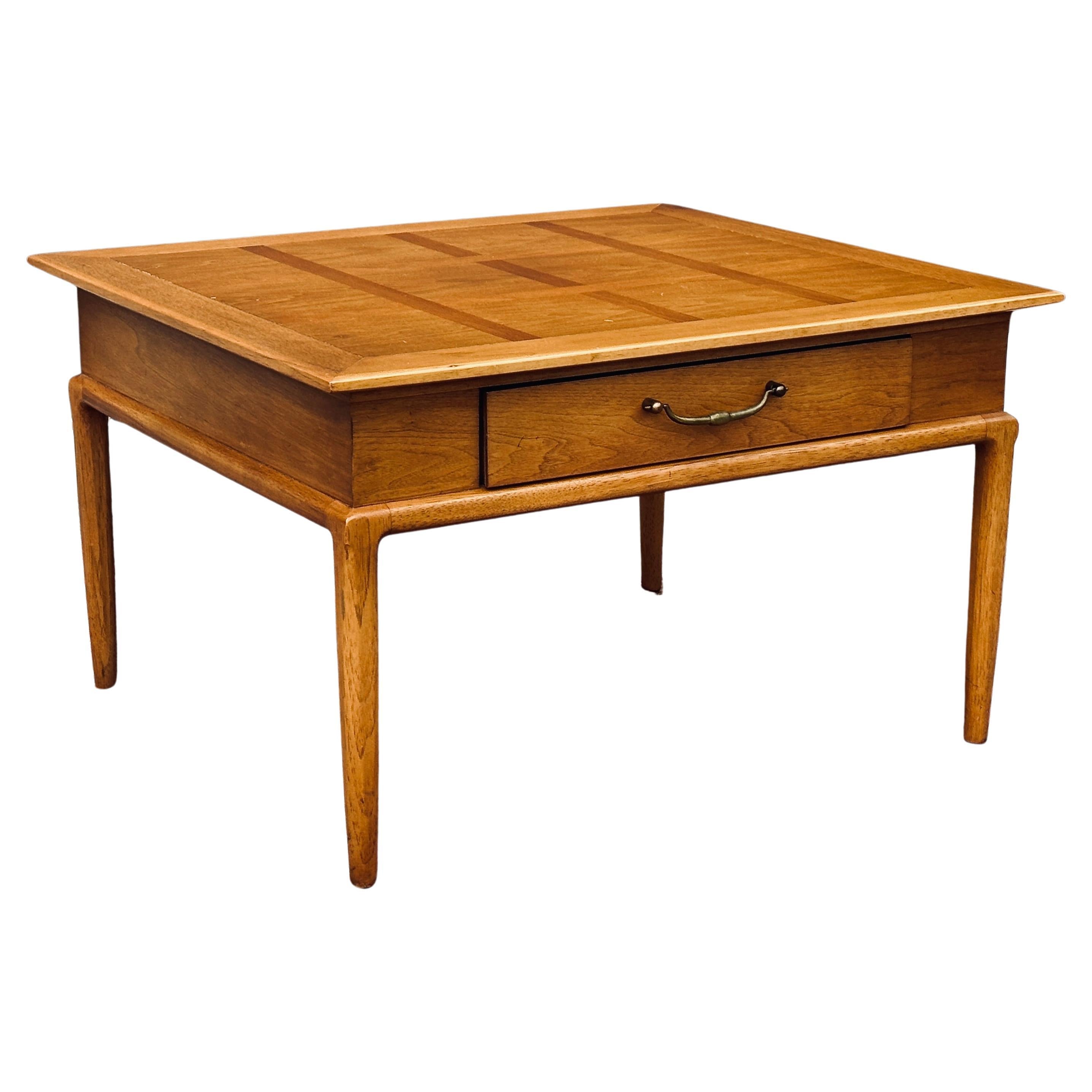The image features a wooden coffee table set against a plain white background, giving it a generic, stock photo appearance. The table is crafted from light brown wood and showcases a detailed inlay on its surface, featuring a rectangular pattern with alternating darker and lighter bands forming a checkered design. It stands on four plain but rounded legs, with the tabletop slightly overhanging the drawer box, which is located on the long side of the table. This drawer is adorned with a simple yet elegant brass pull handle that has a few decorative details. The overall construction and finish of the table emphasize the wood's natural texture and craftsmanship, giving it a timeless and antique appeal.